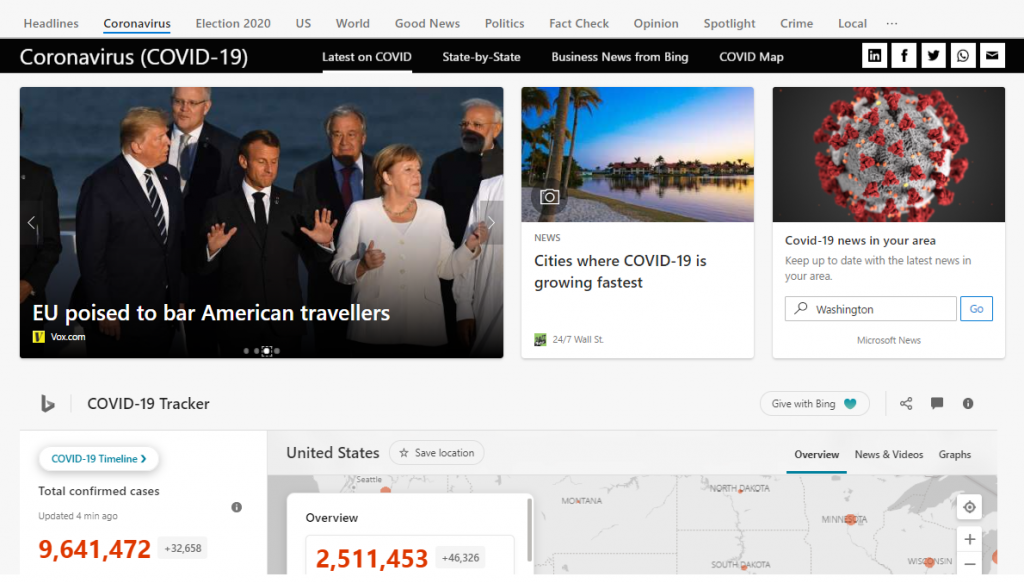In this intricate and multifaceted image, various elements converge to depict a dynamic scene influenced by the ongoing COVID-19 pandemic and its global implications. Prominently featured is the portrayal of business news being disseminated across major social media platforms, including LinkedIn, Facebook, and Twitter, illustrating the interconnectedness and rapid spread of information. 

In the foreground, online students engage interactively, some with hands raised, symbolizing continuous education in the era of remote learning. To the side, a group of politicians and members of the European Union are shown deliberating, poised to make crucial decisions such as barring American travelers in response to the escalating health crisis, an issue further discussed on Vox.com.

The background composition incorporates urban elements with cities experiencing fast-growing COVID-19 cases depicted against a clear blue sky, interspersed with the serene elements of nature such as water, sand, gravel, and flowers, suggesting a contrast between the calm environment and the turbulent state of global affairs. 

Additionally, a COVID-19 tracker prominently displays the real-time frequency of updates, showing a staggering total of 9,641,472 cases, with a recent daily increment of over 200 users and a total of 2,511,452 new cases. Specific states like Texas, Washington, Montana, Minnesota, and Wisconsin are mentioned, providing a localized aspect of the outbreak's impact. 

The overall scene is a blend of contemporary life, underpinned by the themes of news dissemination, education, political action, and the pervasive influence of the COVID-19 pandemic, encapsulating a moment of historical significance.